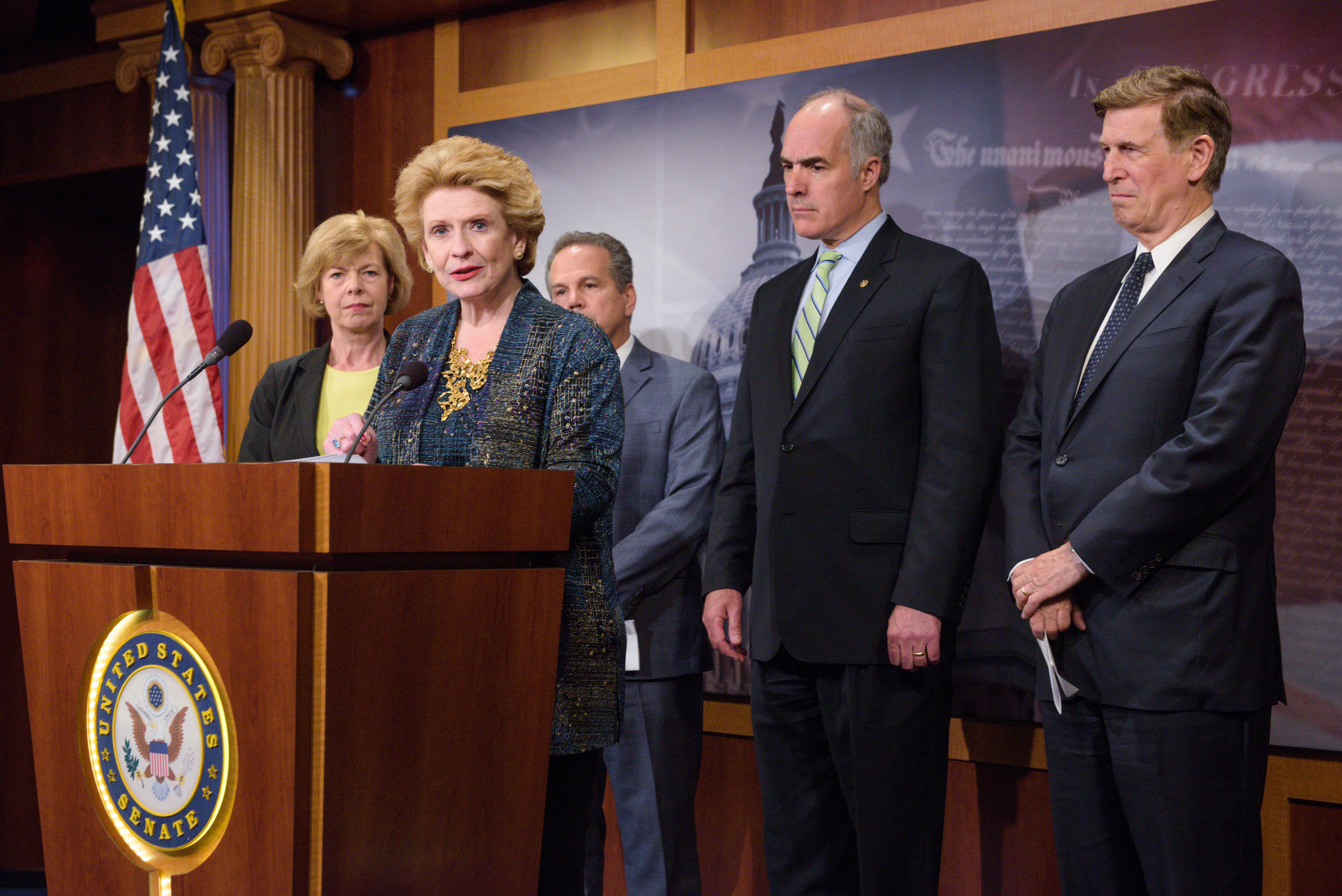The photograph captures a solemn news conference at the United States Senate, featuring a diverse group of individuals in a formal setting. At the front, a wooden podium, adorned with the United States Senate seal prominently displaying an eagle, anchors the scene. Positioned at the podium's black microphone is a serious-looking woman with golden-brown hair, wearing a distinctive blue suit jacket with gold accents over black pants.

Flanking the podium, a United States flag stands draped to the left, and a row of three men and another woman are aligned behind the speaker. The second woman, with short blonde hair, is dressed in a black blazer over a white blouse and stands to the speaker's left. To the speaker's right, the first man wears a blue suit and a blue-yellow striped tie, distinguished by his gray hair and a small lapel pin. Next to him, another man with medium brown hair dons a blue suit, while the third man’s attire remains less distinct but equally formal. In the background, a majestic room with Greek columns and patriotic imagery, including a backdrop depicting the Capitol Dome and historical documents, completes the setting. All individuals present exude a stoic demeanor, underscoring the gravity of the event.